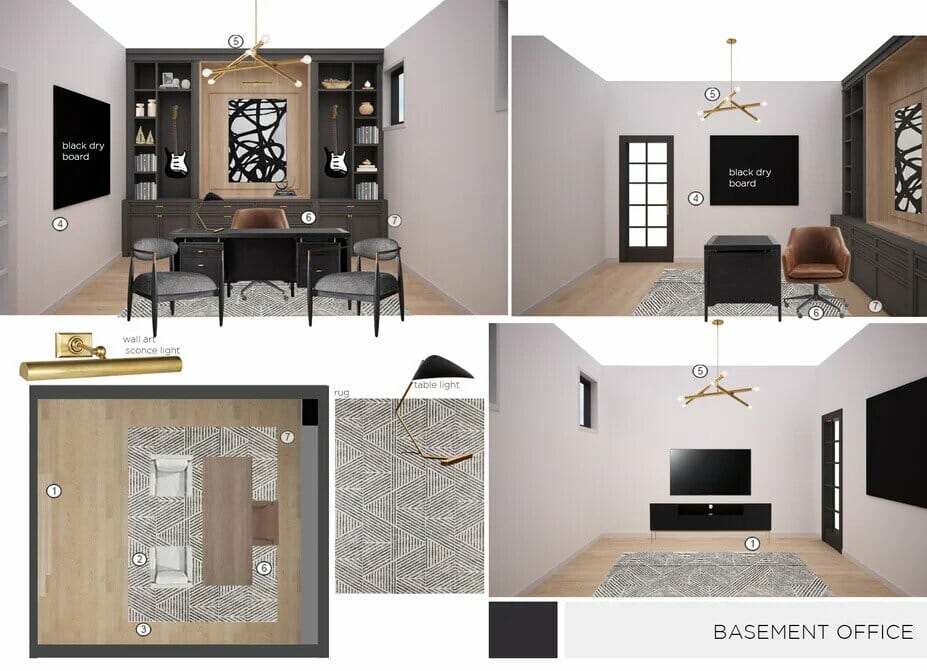The image is a collection of four computer-generated visuals showcasing various perspectives of a "basement office" setup in progress. 

**Top Left:** This view presents a completed room with a black desk, accompanied by a chair behind it and two smaller chairs in front. A bookcase stands behind the desk, while a black square—possibly a poster or monitor—adorns the left wall. Centered above is a light fixture.

**Top Right:** This angle offers a different perspective of the same office. It features the back of a desk chair in the foreground and a brown chair to its right. The far wall exhibits the black poster or monitor seen earlier, positioned to the left of a door, while a ceiling fan hangs from above. Cabinets line the right wall, which changes color above these storage units.

**Bottom Left:** An aerial schematic view of the room reveals a wooden floor and a black-and-white carpet with angular striped patterns. The arrangement includes two white chairs and a desk. A brown bar with some text appears above this schematic.

**Bottom Right:** This final room view highlights light gray walls, a wooden floor, and an area rug with black-and-white designs. A black stand supporting a monitor or TV sits against the far wall, and a ceiling fan is visible. The left wall has a window, while the right wall features a door with a black poster or monitor adjacent to it. Below this image, the words "basement office" are written inside a light gray rectangle next to a black square.

In summary, the images collectively illustrate different stages and perspectives of setting up a monochromatic-themed basement office, complete with furnishings, wall decor, and floor patterns.